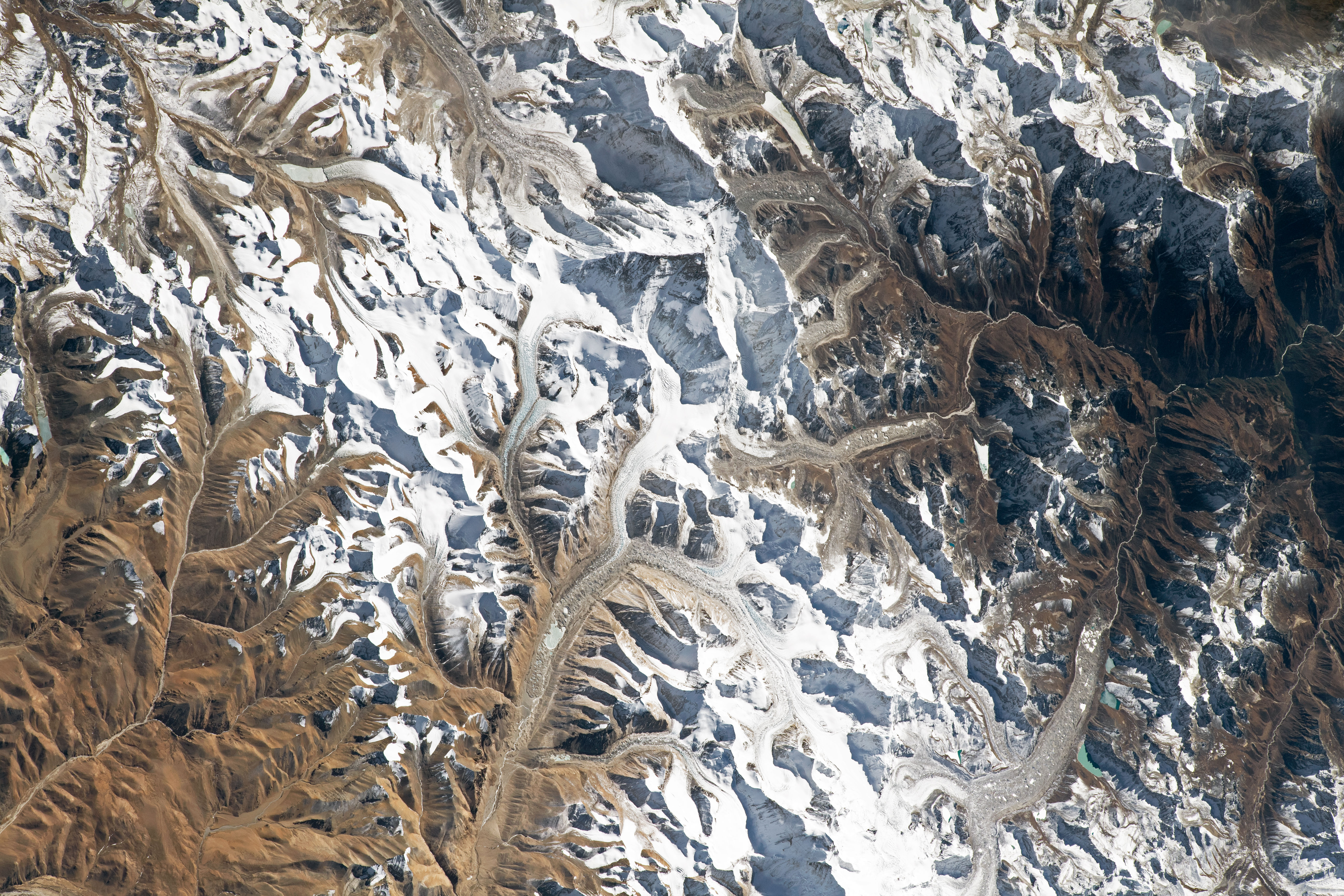The image is a rectangular, top-view photograph that is wider than it is tall. The scene captures a winter landscape from a high altitude, displaying the intricate details of snow-covered terrain with underlying natural elements. The ground, blanketed in snow, shows various shades of white, blue, and brown. Brown tones represent leaves, roots, and possibly plant stems frozen to the ground, branching out from the bottom left corner to the right side of the image. Blue tinges give a cold, icy feel to the landscape, indicating the frigid temperatures and frozen state of the vegetation. The background is primarily gray, intertwined with brown and white, and faint bluish hues, suggesting an overcast winter sky. The photograph focuses on how snow and ice affect the natural environment, particularly the plants, after a snowstorm. The quality of the image is detailed enough to discern these features clearly, and there is no text present in the photo.